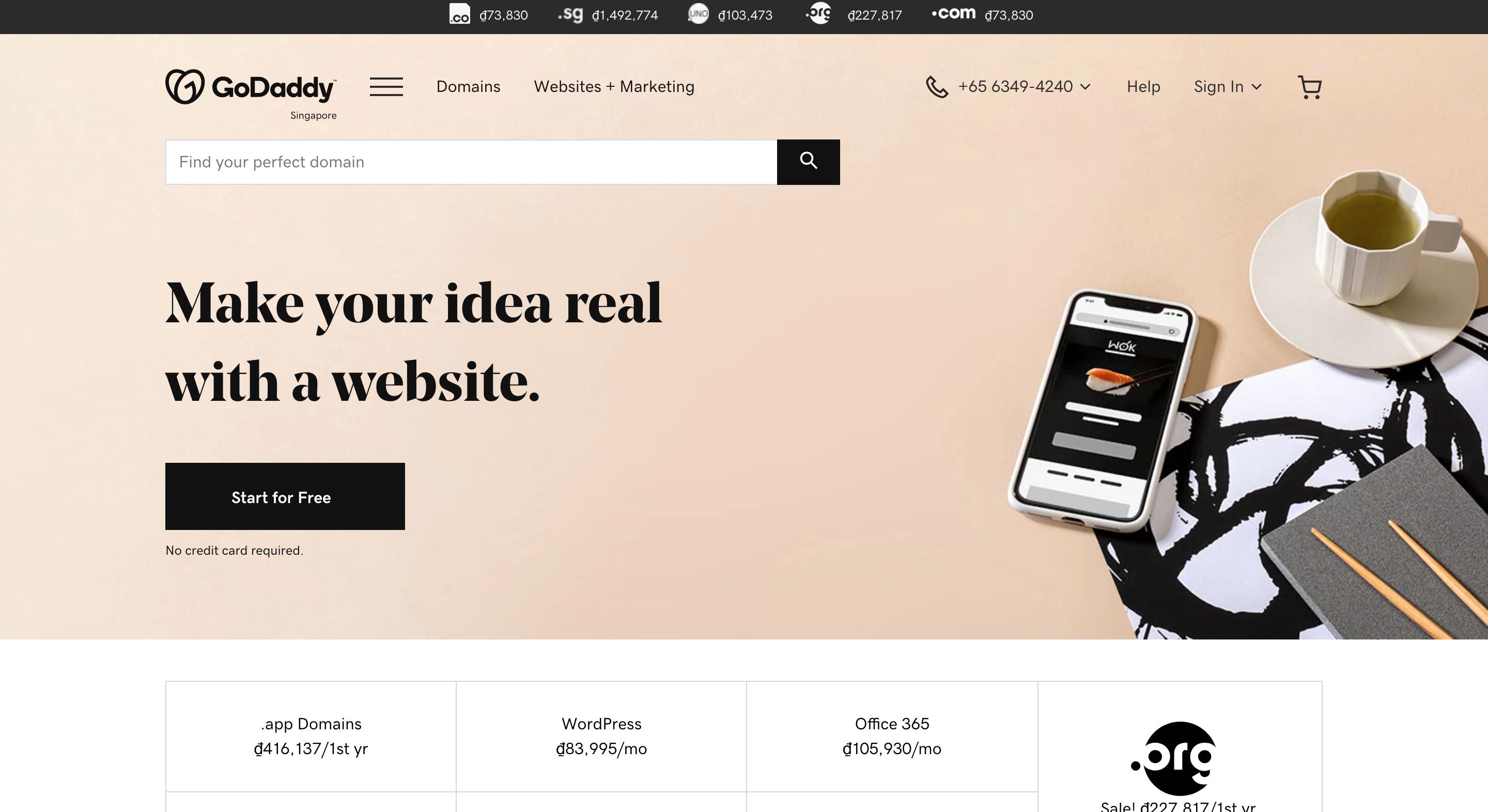This image captures a screenshot of the GoDaddy homepage. Prominent tabs for navigation are visible, including "Domains," "Websites," and "Marketing," along with options for "Phone Number," "Help," and "Sign In." A prominent search bar is present, accompanied by the slogan "Make your idea real with a website. Start for free, no credit card required." 

Near the bottom, various service packages are listed, featuring unclear metrics: "App Domains - $4.16 first year," "WordPress - $8.39/month," and "Office 365 - $10.59/month." The bottom right corner highlights a ".org" domain option.

The visual aesthetic of the page includes a light beige background with black text. Accessories in the right-hand corner of the scene include a coffee cup on a saucer, a grayish-white smartphone, and a black notebook. The notebook appears to have either chopsticks or drumsticks resting on a gray book placed beneath it.